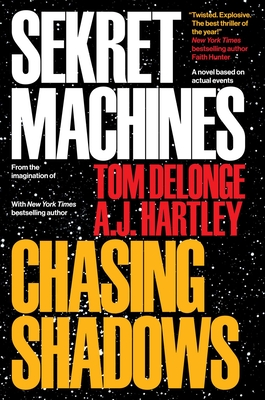This is a highly detailed poster for the book titled "Sekret Machines: Casting Shadows." The background is predominantly a space scene, filled with twinkling stars set against the vastness of a black night sky. The title "SEKRET MACHINES" is prominently displayed in bold white letters, occupying approximately the top third of the poster. Above the word "MACHINES," there is an intriguing tagline that reads, "A novel based on actual events."

At the bottom third of the poster, the subtitle "CASTING SHADOWS" is presented in all uppercase font, commanding attention. Centered in the middle right portion of the poster, the names "Tom DeLonge" and "A.J. Hartley" are stacked vertically in striking red letters. 

To the left of the authors' names, another line reads, "From the Imagination of Tom DeLonge and New York Times best-selling author A.J. Hartley," providing context about the collaborative nature of this work.

In the upper right-hand corner of the poster, an endorsement quotes New York Times best-selling author Faith Hunter, exclaiming, "Twisted. Explosive. The Best Thriller of the Year!"

This intricately designed poster captures the mysterious and thrilling essence of the book while highlighting the notable figures involved in its creation.